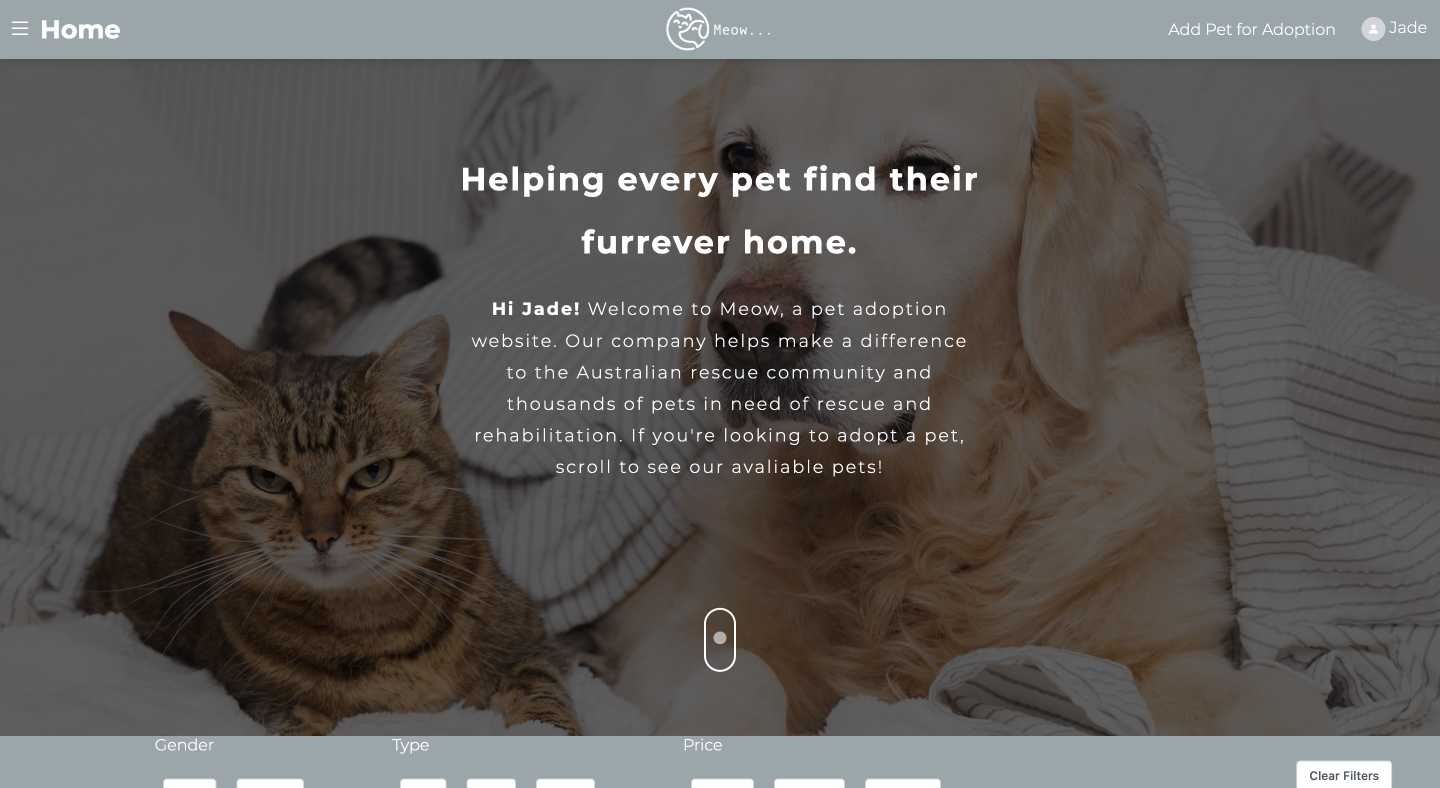This is a detailed and cleaned-up caption for the given image:

---

The web page for "Meow," a pet adoption website, prominently features a warm and inviting layout designed to help pets find their forever homes. At the very top center of the page, there is an endearing logo depicting a drawn cat and dog next to the word "Meow." 

In the upper left corner, a "Home" button accompanied by a three-stripe menu icon provides easy navigation. On the opposite side, in the upper right corner, there is an "Add Pet for Adoption" link, alongside a user icon that indicates the presence of a logged-in user named Jade.

Dominating the center of the page is a heartwarming image featuring a serene adult golden retriever cozily covered with blankets and a small, tiger-striped house cat with green eyes resting beside it. Overlaying this image, the phrase "Helping Every Pet Find Their Furrever Home" is prominently displayed, with "furrever" playfully spelled to emphasize the site's mission.

Below this motto, a personalized greeting reads, "Hi Jade, welcome to Meow, a pet adoption website. Our company helps make a difference to the Australian rescue community and thousands of pets in need of rescue and rehabilitation. If you’re looking to adopt a pet, scroll to see our available pets."

Finally, at the bottom of the page, there are options labeled "Gender," "Type," and "Price," allowing users to filter and select the type of pet they wish to adopt, ensuring a seamless and user-friendly experience.